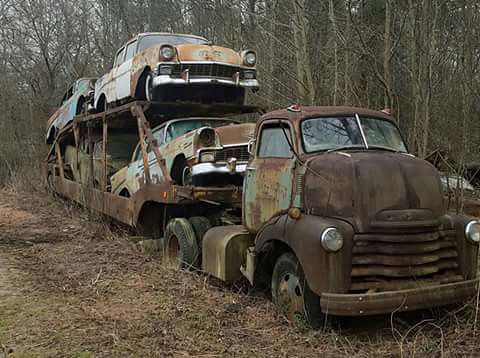This photograph features an old, abandoned car carrier truck parked in a desolate, woodland area, surrounded by leafless trees with varied shades of brown trunks. The truck appears to be a vintage Ford semi from the 1930s or 1950s with a rounded cab, rounded nose, and small windows. The heavily rusted truck, once green in parts, showcases a large fuel tank on its side and wheels sunk into the dirt of a dark brown, withered grass field. Behind the truck, a two-deck car carrier trailer holds four cars from the 1950s, each in various stages of rust and disrepair. The colors of the cars range from cream to blue to rust-brown, with one showing terracotta hues. Some chrome details on the vehicles still manage to shine. Despite the truck’s dilapidated state, its windows remain intact, though its tires are deflated. The gray sky overhead amplifies the abandoned and forlorn atmosphere of the scene, with a hint of white in the background that may be snow.